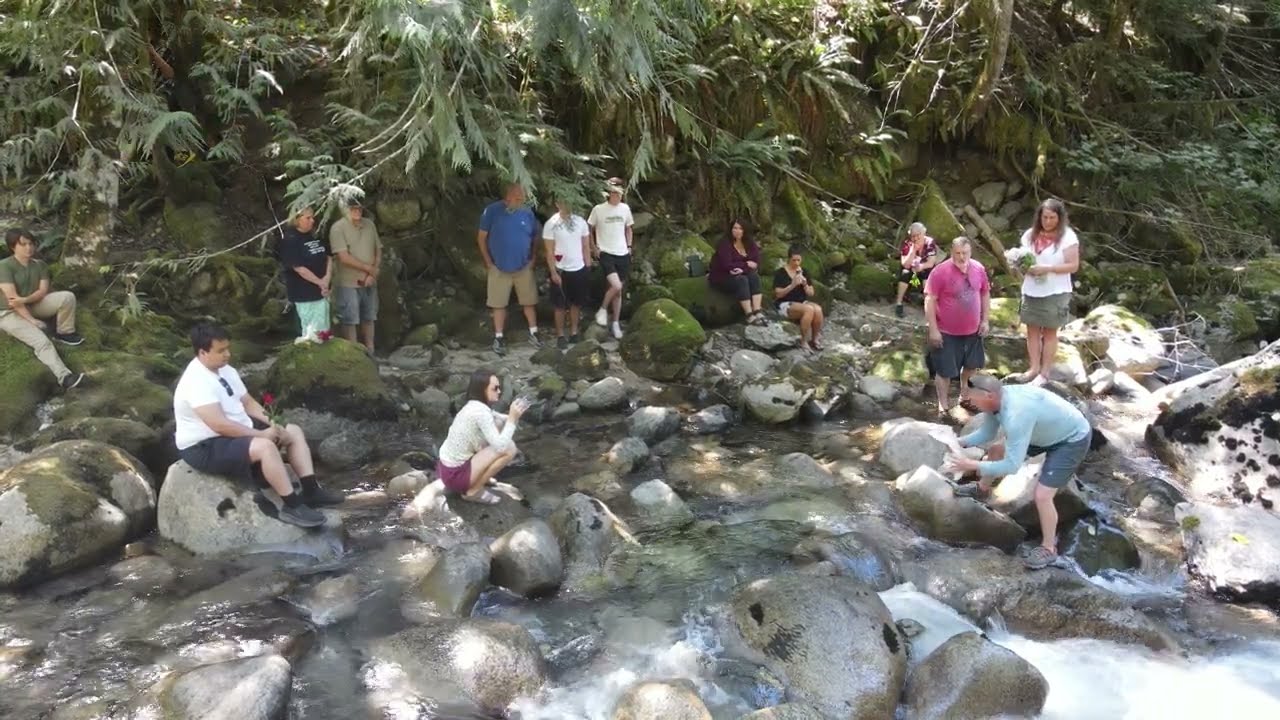The image depicts a lively scene by a stream with water cascading over rounded stones. A large gathering of about 10-12 people is evident, with individuals standing at the edge of the water, immersed in the stream, and positioned along the sides on rocks. They are all attentively focused on a man towards the right side of the image. This man is wearing a light blue top and gray shorts and has a pair of black sunglasses perched on his head. He is slightly blurred, suggesting movement, and is holding a rock while standing almost at the center of the stream. In the foreground, the stream features both white, frothy water and clear patches where submerged rocks are visible.

To the left, a woman is squatting down, capturing a photo, with a man behind her, identifiable by a red rose and seated on a rock. Another prominent character is a middle-aged woman with glasses, wearing a dark-colored shirt with white patterns and black pants, seated slightly towards the back. 

The surroundings are lush with vegetation, featuring overgrown trees, green moss on the rocks, and broad leaves sprouting from larger rocks. Tree branches hang down from the upper left corner, framing the top of the image with greenery. Numerous other persons dot the scene: a person in a green t-shirt and tan pants, someone in a white t-shirt and black pants sitting directly on a rock, another woman in a white shirt and purple shorts actively engaged in photography, and several others in a mix of casual attire including dark clothing and shorts. 

The rocky terrain varies in color from grayish-tan to brownish where wet. Large logs and tree trunks intersect the scene, adding to the natural, untamed beauty of the setting. The group generates a sense of camaraderie as they gather in this picturesque and dynamic stream environment, perhaps united by a shared interest or familial connection.